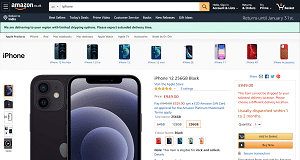The image depicts a screenshot taken from the Amazon Australia website (amazon.co.au) on a smartphone. The user appears to be viewing a product page for the iPhone 12, specifically focusing on the black color variant. The product is rated five stars, although the exact number of ratings is difficult to discern from the image. The available color options displayed include black, red, teal, green, and a pinkish hue. 

On the left side of the page, there are thumbnail images of the iPhone, including a video thumbnail that offers a detailed overview of the product. As you scroll down, the page appears to be partially cut off, but it still shows key details such as a prominent "Buy Now" button in an orange rectangle. Above this is a yellow rectangle, containing text in red, but the specifics are not clearly visible.